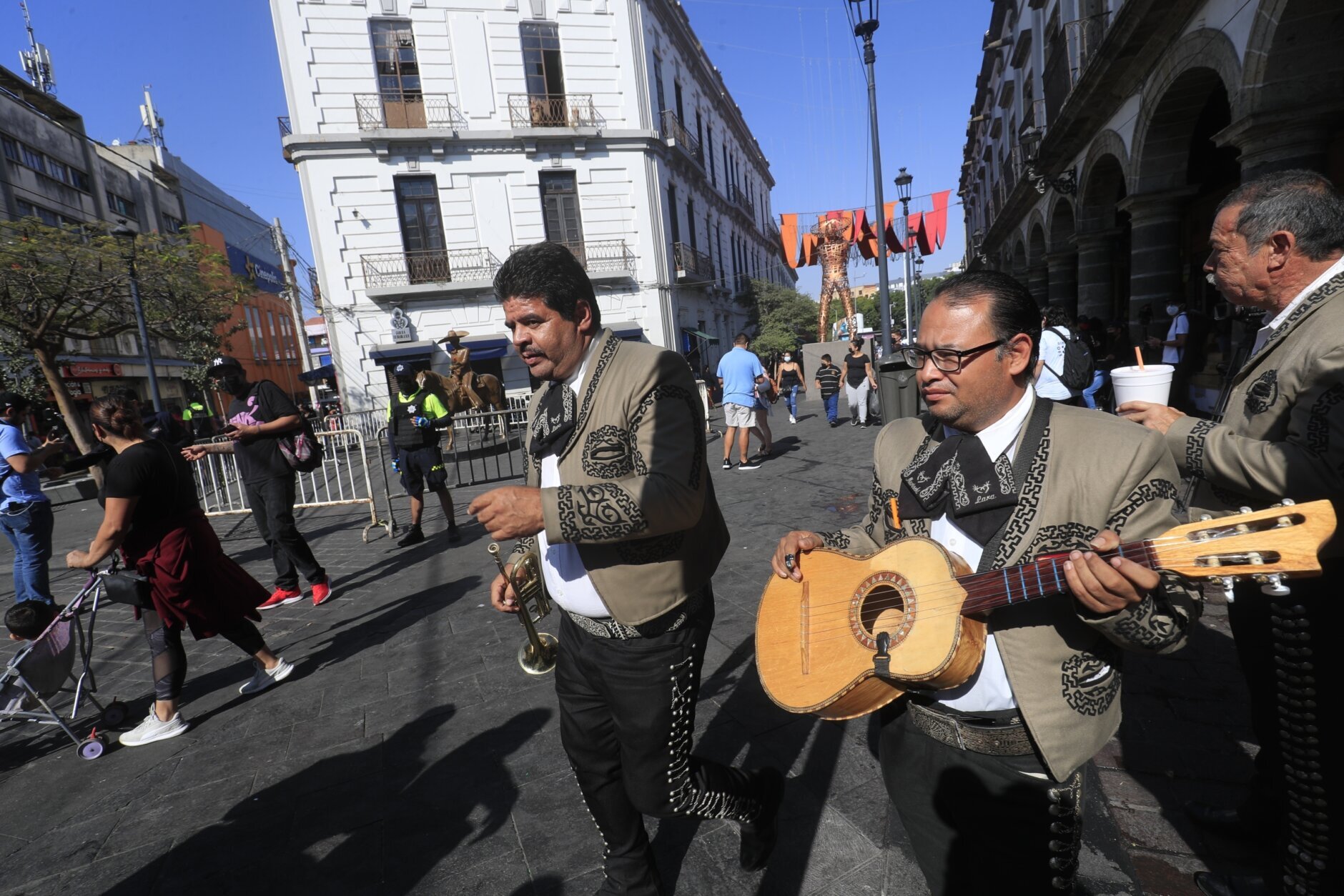In the street scene set on a picturesque brick or cobblestone pavement, likely within a tourist area in a central Mexican town, stands a mariachi band taking a well-earned break. The trio, attired in striking costumes featuring black pants adorned with intricate designs, short blazer-type jackets over white button-down shirts, and black bow ties, catches the eye. The leftmost gentleman, holding a trumpet, stands beside the middle member, a shorter man with glasses cradling a small guitar. To their right, the third member, slightly taller and heftier, enjoys a drink from a styrofoam cup with a contented smile. The bustling background displays a harmonious blend of historical and lively elements, including several multi-story buildings—none towering beyond four stories—featuring an old white building and an arched structure. People wander by, families with children in tow, capturing a vibrant, sunny day under a clear blue sky. A lady pushes a carriage in the left side of the frame, while red flags hanging on clotheslines flutter near a bronze statue, contributing to the scene's vivid tapestry of life and culture.